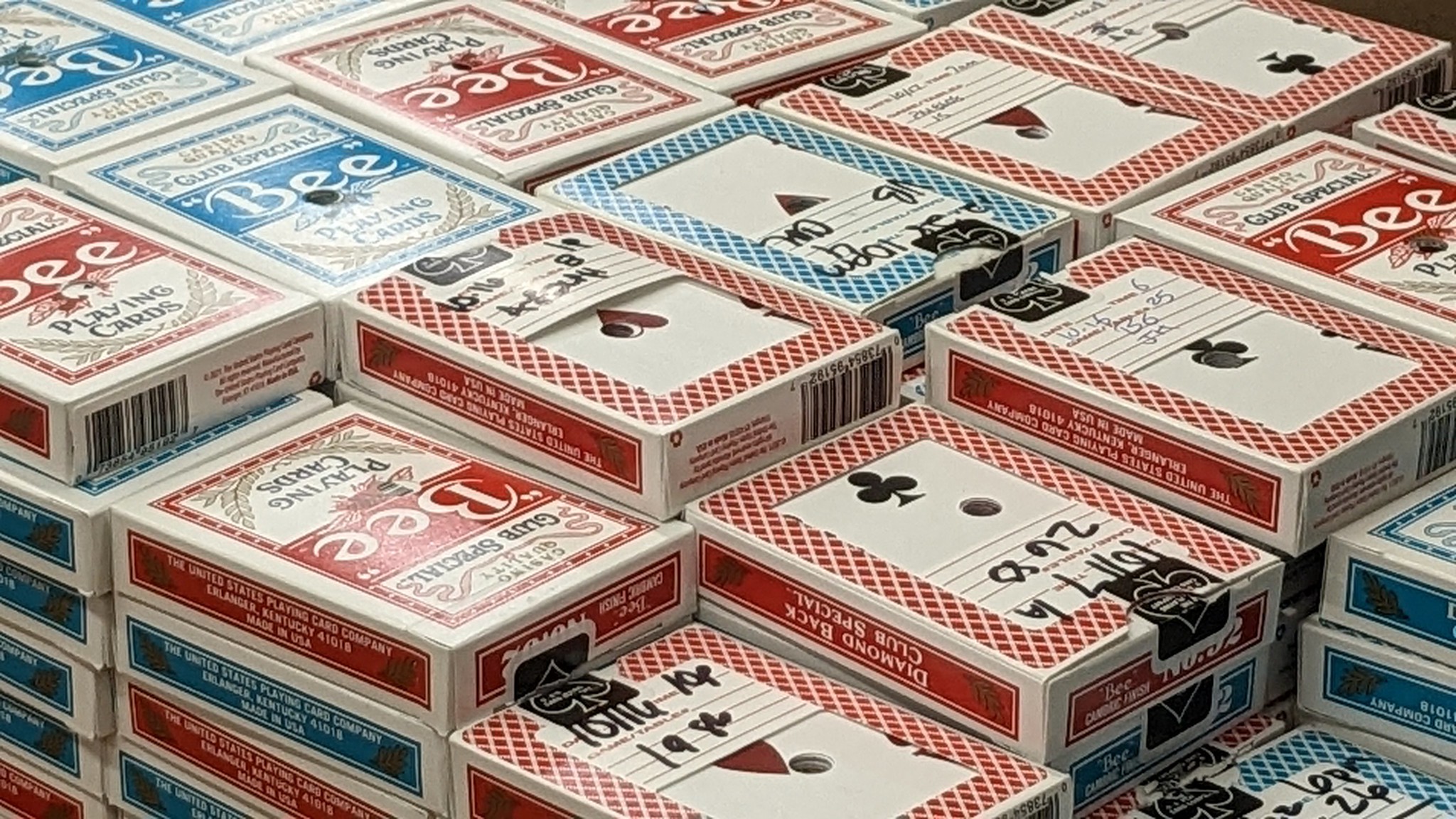Below is a cleaned-up and highly detailed caption for the image:

---

The image showcases a vast assortment of playing card decks, neatly arranged in stacks that suggest an organized collection or inventory. These decks come in two distinct color variations—blue and red—and belong to a brand identified by the letter "B" prominently displayed on the packaging in large, bold font. The design of the packaging exudes a vintage charm reminiscent of styles from the 1940s or even earlier, adding a touch of classical elegance.

The numerous decks are arranged in a structured manner, with the stacks forming what could be several layers, possibly up to seven. Some of the decks are adorned with stickers displaying dates and numbers, indicating a possible cataloging system. One sticker reads "10-16-1986," which might signify the date the deck was acquired, while another displays "2680," the meaning of which is less clear but suggests a form of identification or batch numbering. The stacks are packed closely together but not overly tight, allowing for some slight looseness at the top layers.

The overall impression is one of abundance, perhaps filling a small pallet or tote, but the focus remains solely on the decks of cards, giving the viewer a sense of the sheer volume and meticulous organization of this card collection.

---

This detailed caption provides a vivid and comprehensive description of the image, enhancing the viewer's understanding and appreciation of its contents.